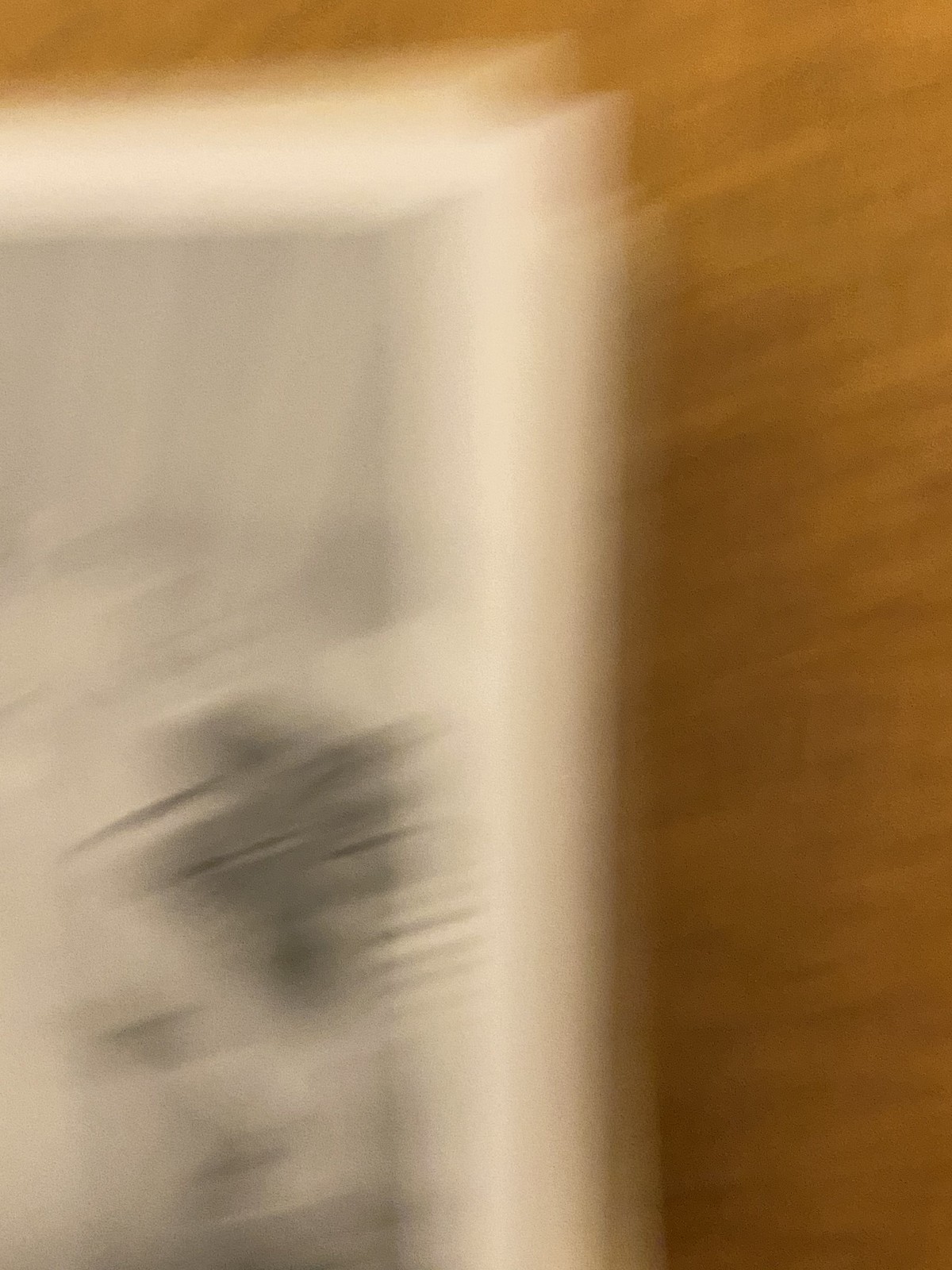This color image is very blurry and out of focus, making it difficult to accurately identify the subject. The photo appears to be a close-up shot of a scene with a brown vertical surface, which could be a wall. To the left, starting from the middle of the image and extending upward, there is a white, somewhat thick frame-like object that bends 90 degrees to the left at the top. Inside this white border, there is a gray section that may contain some form of sketch or artwork, displaying various shades of black, gray, and white. The image quality is extremely poor, with grainy, elongated lines across it, which may be due to camera movement or poor device quality. The photo does not contain any people, animals, plants, signs, buildings, or motorized vehicles.